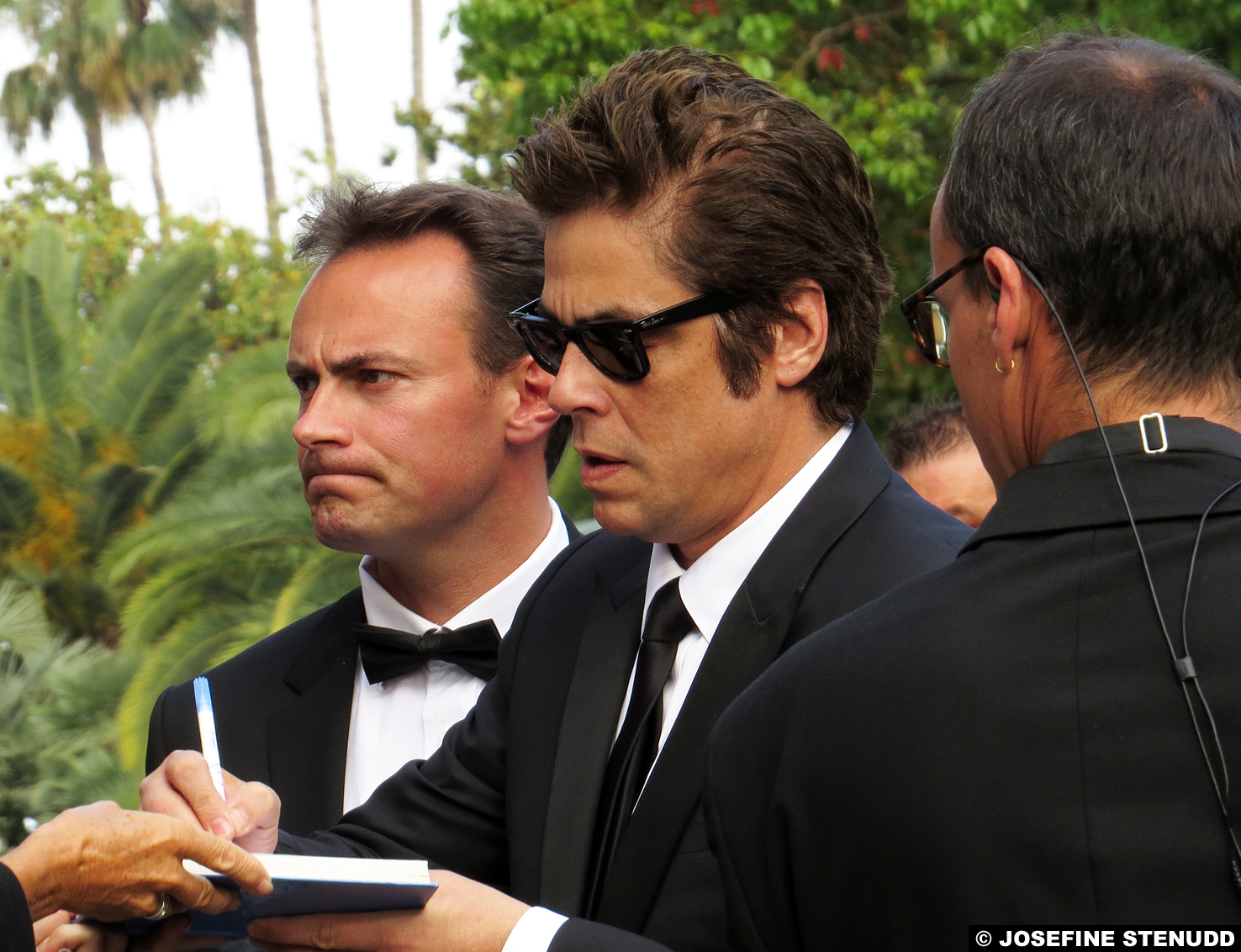The photograph captures a candid, wide rectangular outdoor scene featuring three men dressed in formal black suits. The man on the right, with his back to the camera, sports a black suit and sunglasses, his head tilted slightly to the left, revealing an earpiece and a gold hoop earring. To his left, directly behind him, stands Benicio del Toro, identifiable by his thick brown hair and somber expression, also clad in a black suit with a white shirt and dark tie. He is engaged in signing an autograph on a white stack of paper held by a woman, her hand adorned with a ring extending into the bottom left corner of the frame. The third man, to the left of Benicio, wears a black tuxedo with a bow tie and a white shirt, staring off to the side with a serious demeanor. The backdrop features a bright sky obscured by radiant sunlight, casting the surrounding trees—some with green foliage and others with red, yellow, and orange leaves—in a vivid, almost ethereal light.